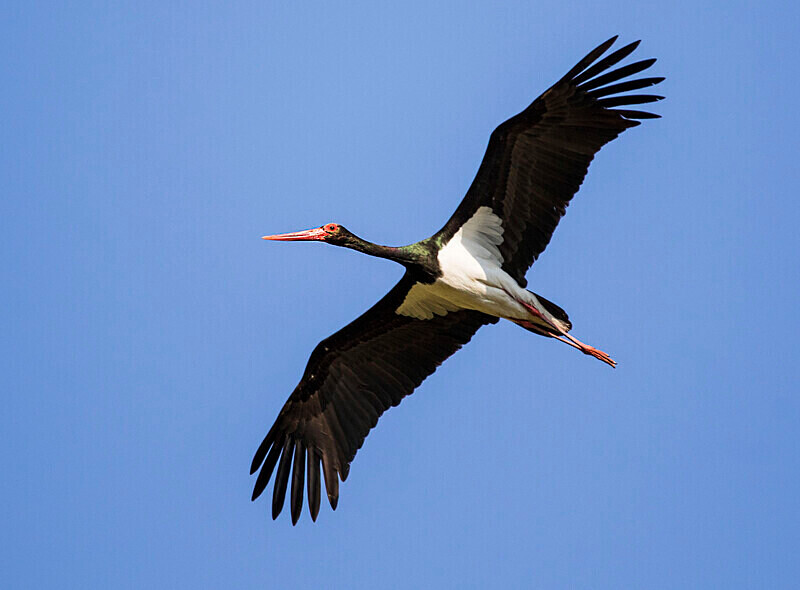This photograph captures a black stork in mid-flight against a clear, vivid blue sky. The stork dominates the frame with its impressive wingspan, fully outstretched. The underside of the bird reveals detailed features: striking black wings with distinct feather tips, a contrasting white underbody, and long red-orange legs trailing behind. Its elongated neck, sheened with tinges of green and purple, leads to a sharp red-orange beak and eyes surrounded by a reddish hue. The sky is uniformly blue, devoid of clouds, emphasizing the bird as the focal point of the image in a tranquil, mid-flight glide.